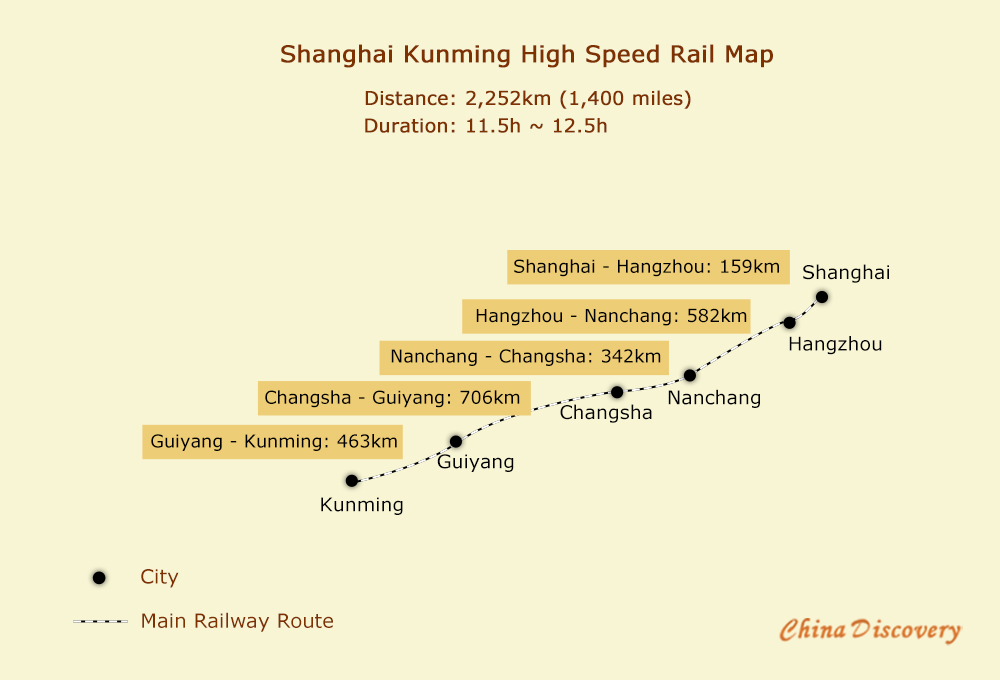The image illustrates a "Shanghai-Kunming High-Speed Rail Map" set against a beige-pink background. The total distance covered by this high-speed railway is 2,252 kilometers (1,400 miles), with a travel duration ranging from 11.5 to 12.5 hours. The rail line is depicted as a dotted route with black dots indicating key cities: starting from Kunming on the left, followed by Guiyang, Changsha, Nanchang, Hangzhou, and finally Shanghai. Additionally, rectangular yellow labels are placed between cities to specify distances, such as "Guiyang to Kunming, 463 kilometers" and "Shanghai to Hangzhou, 159 kilometers." There is a key at the bottom of the map explaining that black dots represent cities and dotted lines mark the main railway route. This map is part of a "China Discovery" series, detailing this critical high-speed rail network route.